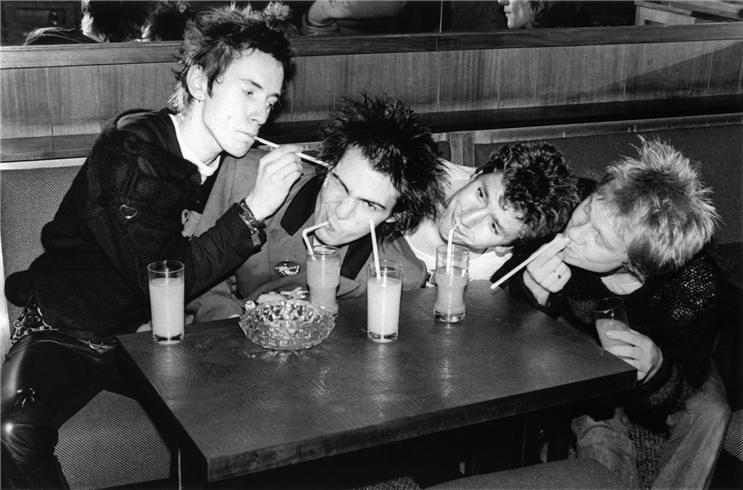In this charming black and white photograph, four young men, resembling mod rocker musicians from several decades ago, gather in the booth of an American-style diner. The image, possibly staged given its timeless feel, captures their mischievous energy. A thick, rectangular wooden table occupies the foreground, topped with a crystal ashtray and four beverages in clear glasses, all equipped with straws — except for one on the left. The man on the far left, drinkless of straw, playfully inserts his straw into the ear of the man next to him, who grimaces while sucking on his own straw with one eye squeezed shut. The two men on the right join the fun, each engaging with their straws, twisting their mouths, and grinning. In the background, wood-paneled boards frame the scene, enhancing the nostalgic ambiance. The laughter and camaraderie of the moment suggest these friends are thoroughly enjoying each other’s company, making the photograph both endearing and timeless.